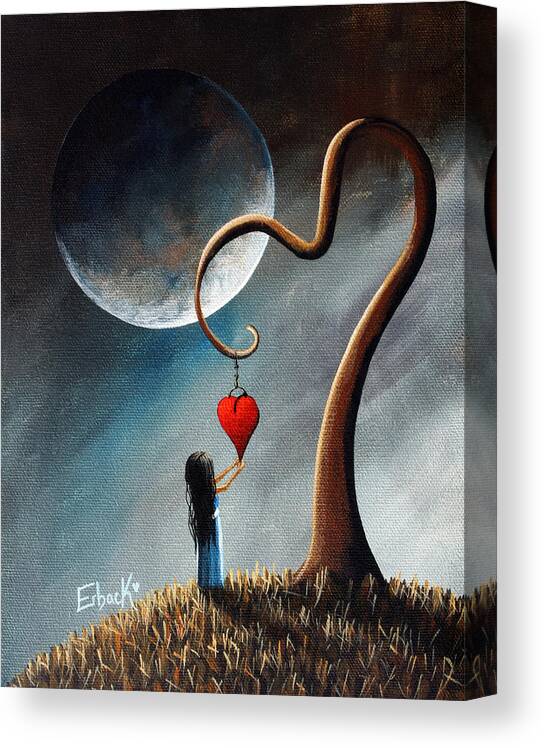The painting, evocative and somewhat melancholy, is meticulously rendered on a thick canvas. It features a somber scene dominated by a dark, stormy sky awash with hues of gray, blue, and purplish-gray. A large, crescent moon, mostly shadowed except for a sliver of white at the bottom, occupies the top quarter of the canvas, casting an ethereal glow over the scene.

In the foreground, a desolate hill covered in brown grass slopes gently, supporting a sinuous, leafless tree branch. The branch, curling and ending in a whimsical hook, suspends a striking red heart. Below, a little girl with long black hair, dressed in a flowing blue dress, stands facing away from the viewer, her arms reaching upward to grasp the heart.

The composition's emotional weight is heightened by the simplicity and barrenness of the tree and the solitude of the girl. The bottom left of the canvas bears the inscription "ERBACK" written in white, possibly the artist's signature, accompanied by a small heart, adding a personal touch to the desolate poetry of the scene.